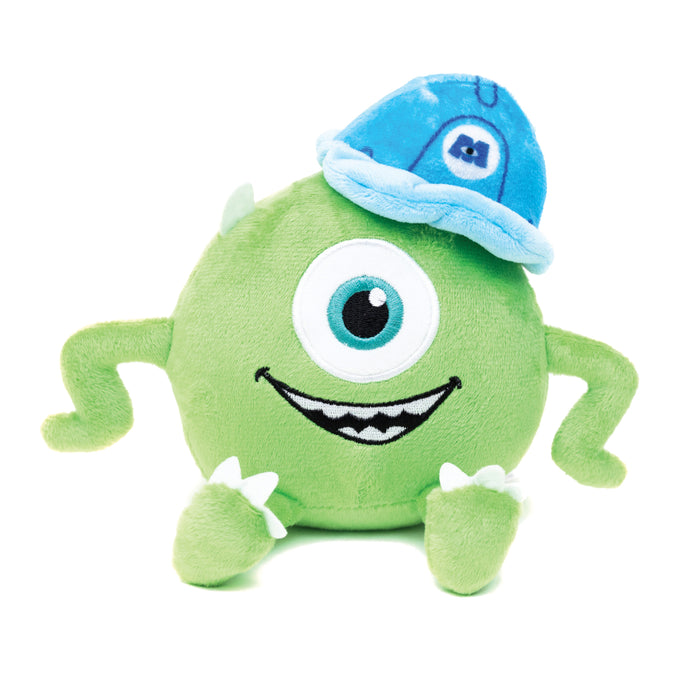This is a detailed product photograph of a plush toy featuring the character Mike Wazowski from the movie series "Monsters, Inc." The plushie is set against a seamless white background and surface, providing a clean, distraction-free view. The plushie depicts Mike Wazowski as a round green figure with a singular large eye that has a blue iris, framed by a big, smiling mouth below. He has two squiggly arms extending from either side of his body, which are possibly posable, given their Z-shaped bends, hinting at internal wiring. His two feet are positioned in front, each adorned with a trio of soft fabric toenails. 

Adding to the character's recognizable features, Mike is equipped with a blue cloth helmet, complete with stitched dark blue lines and the iconic "Monsters, Inc." logo—a white circle with a blue letter "M." The helmet rests on the left side of his head (right side of the image). This meticulously designed plush toy captures the essence of Mike Wazowski, bringing playful charm and a memorable smile to life.